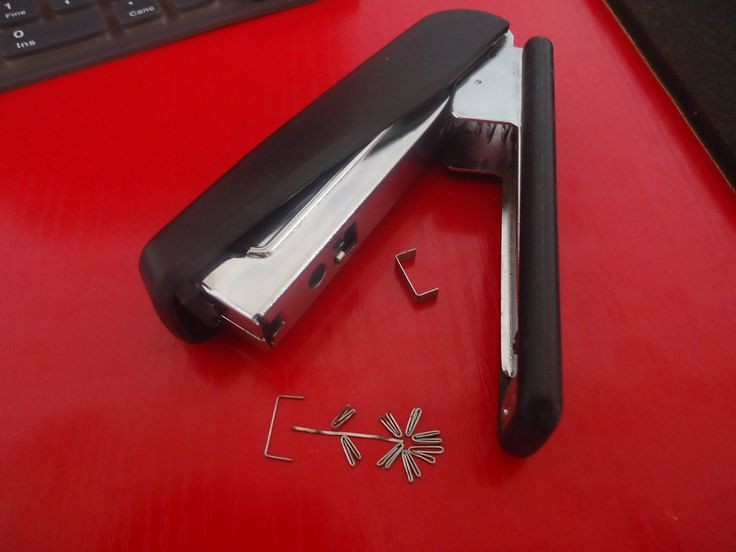The photograph captures a vintage black Swingline stapler lying on its left-hand side atop a bold red surface. The stapler's top, bottom, and base are all black, while the center hinge and interior components display a silvery chrome color. Evident in the scene, several staples have been intricately arranged around the stapler. Some of these staples have been uniquely manipulated to form a display resembling a flower, with an open staple forming the stem, others bent to represent leaves, and the top section arranged to look like the flower itself. The arrangement also includes a small asterisk and an indeterminate symbol, enhancing the creativity of the display. The top-left corner of the image features the bottom edge of a computer keyboard, adding an office context to the scene. The red surface underlines the subjects, providing a striking contrast.